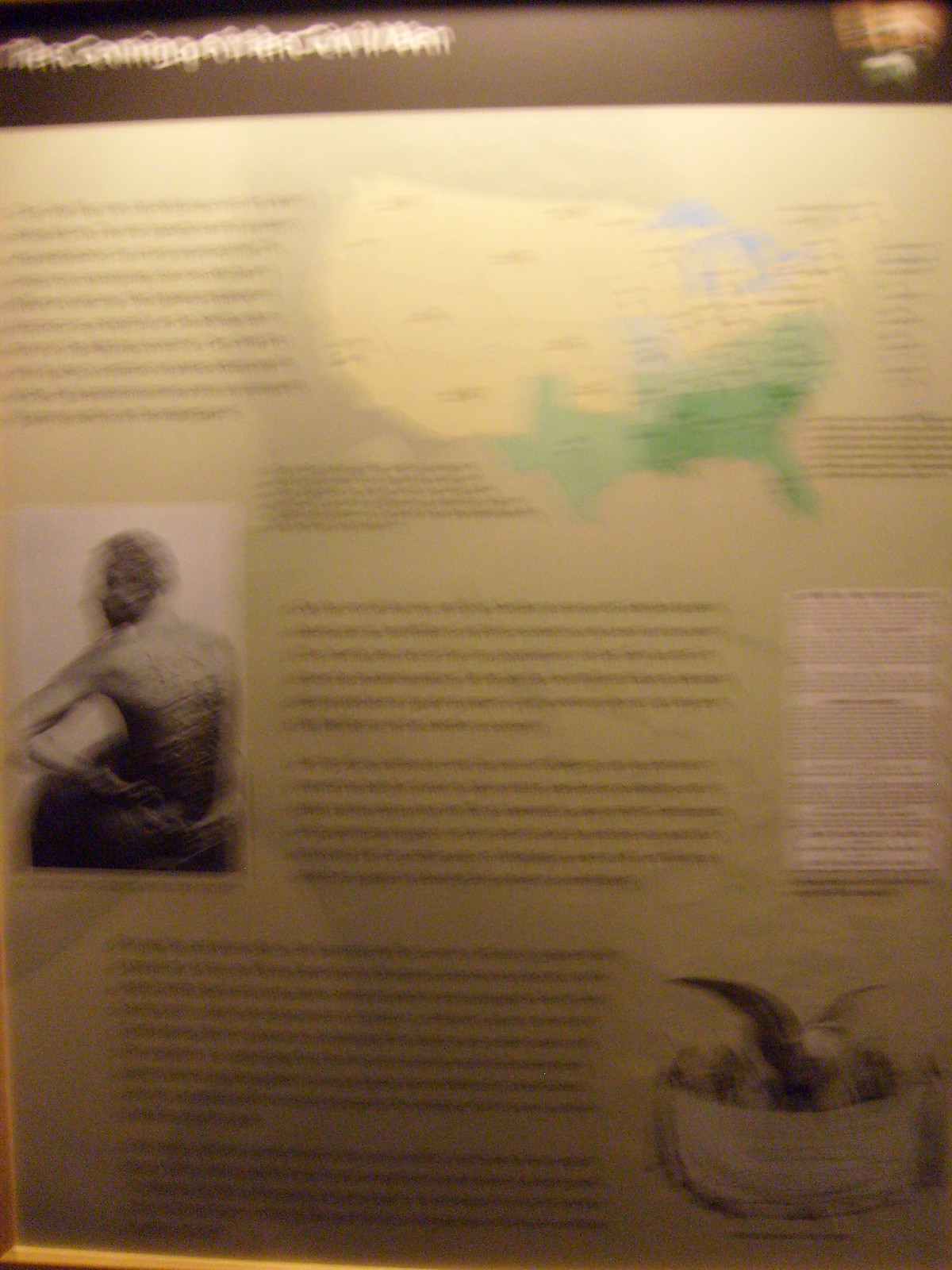This is a photograph of a framed poster mounted on a wall. The image is significantly blurred and out of focus, making details difficult to discern. The frame appears to be a thin strip of yellowish-brown material, possibly wood or plastic, visible in the lower left corner of the image. The poster itself is largely illegible due to its low quality and blurriness.

At the top of the poster, there is a black bar with white text, accompanied by an unidentifiable graphic in the upper right corner. Below this bar, the poster contains a paragraph of black text, alongside a labeled map of the United States. Further down, there is another paragraph of text.

On the left side of the poster, there is a graphic depicting a statue of a man whose back appears to have marks, suggesting he may have been whipped, potentially indicating he is a depiction of a slave. Despite the lack of clarity, the elements and structure of the poster suggest it may be historical or educational in nature.